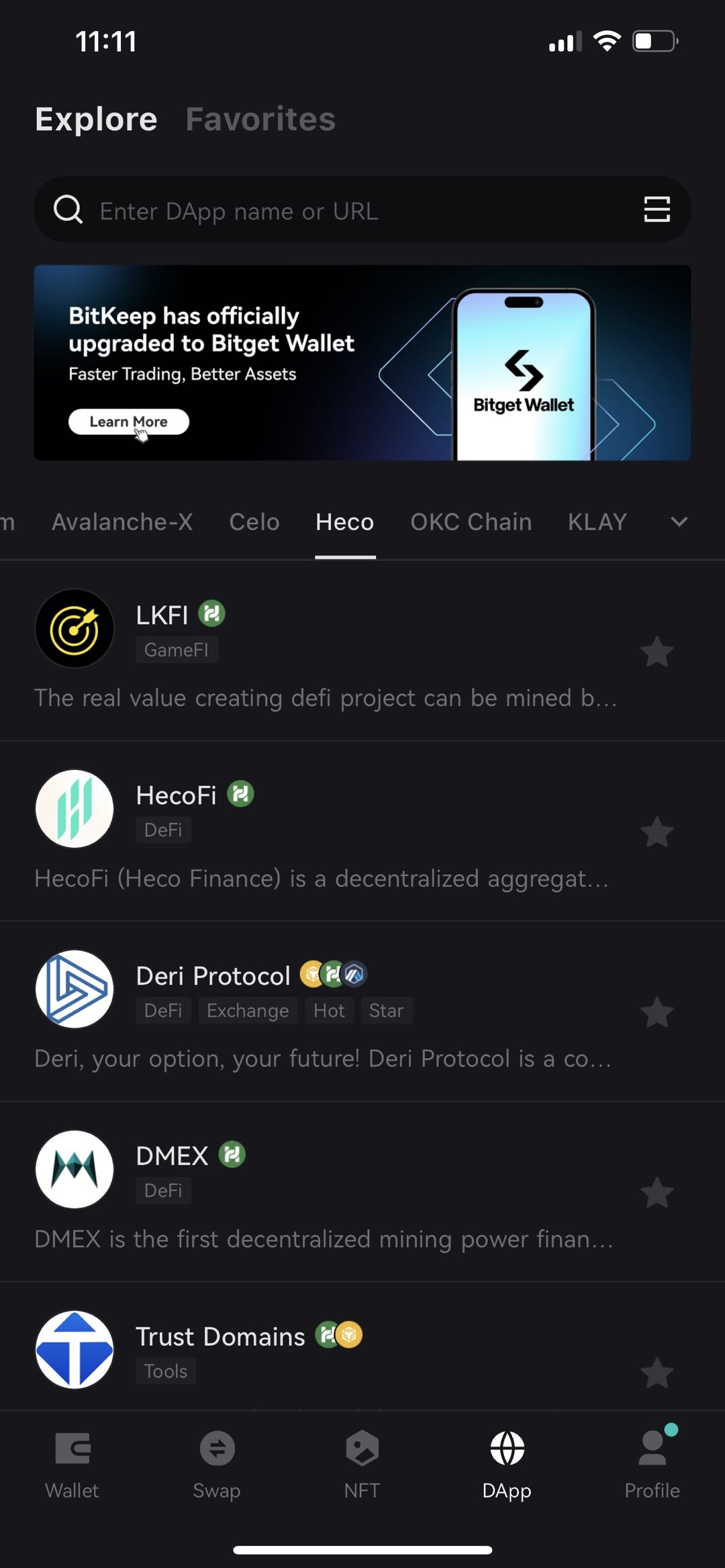This image displays a smartphone screen with various interface elements prominently displayed. In the top left corner, the time is shown as "11:11" in white text. Moving to the right, there are three signal bars and a battery icon showing half battery life.

Below the status bar, two interface options, "Explore" and "Favorites & Highlights," are present, with "Explore" being highlighted. Underneath these, a search bar invites the user to "Enter dApp name or URL."

Following the search bar, there is a prominent advertisement for BitKeep, stating that "BitKeep has officially upgraded to BitGet Wallet. Faster trading, better access." This advertisement features a white button labeled "Learn More" and an image of a smartphone home screen showcasing the BitGet Wallet app.

Continuing down, the screen displays several blockchain network options: Avalanche X, CELO, HECO, OKC Chain, and KLAY, with "HECO" currently selected and underlined.

Below these options, a vertical list of decentralized applications (dApps) on the HECO network is visible, featuring "LFKI," "HECOFI," "Dairy Protocol (DERI)," "DMEX," and "Trust Domains."